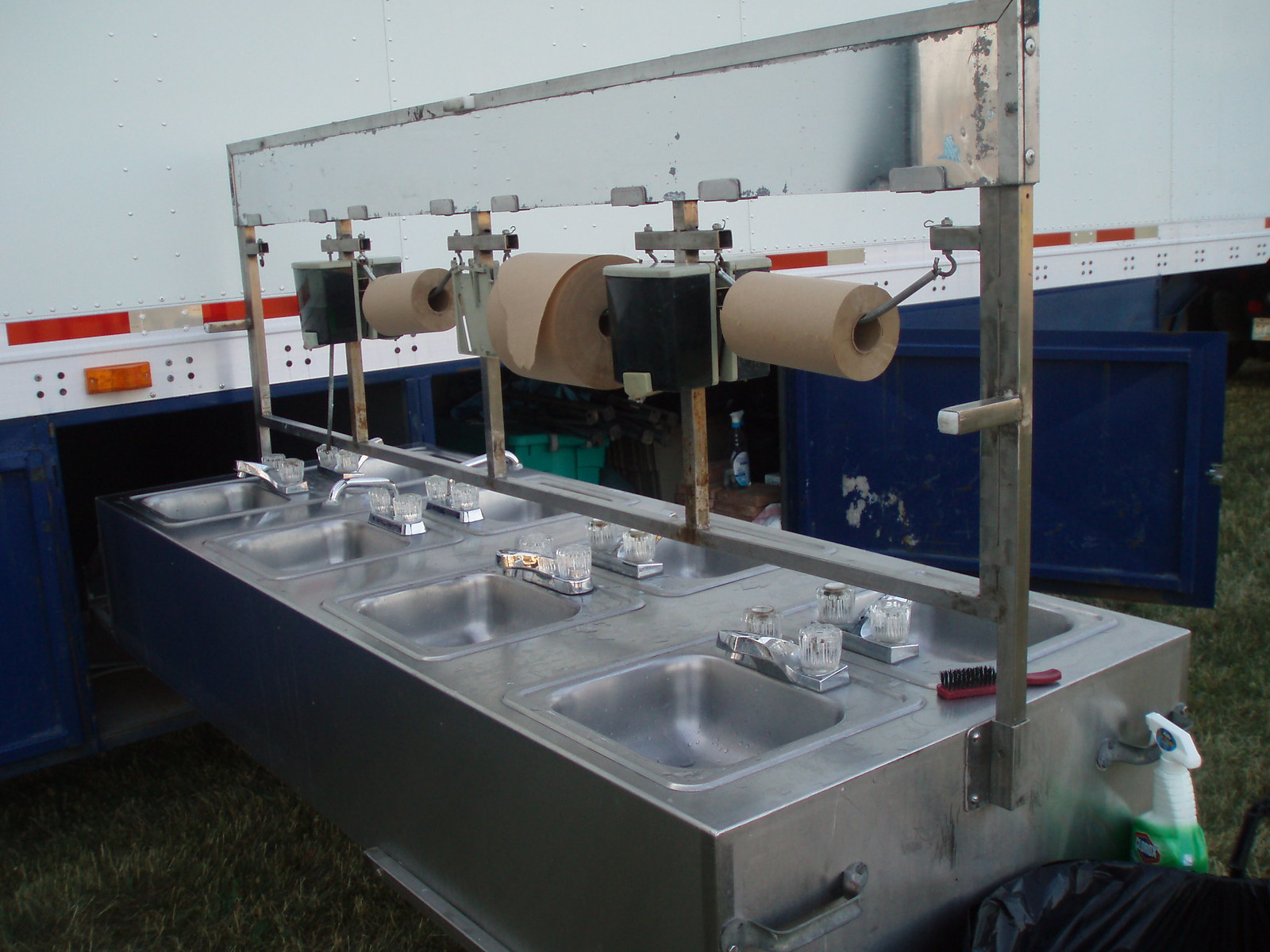The image shows an outdoor, portable washing station, likely situated at a music festival or similar event. The station is attached to a white and blue truck or trailer, with eight metal sinks extending outward. Each side of the elongated rectangular basin features four sinks, equipped with at-home style bathroom faucets. At the center of the station rises a metal frame adorned with soap dispensers and three rolls of brown paper towels. Additional items include a red hairbrush positioned on the right, a white and green Clorox cleaner bottle, and a bit of a black trash bag peeking out on the far right. The backdrop reveals a grassy area, reinforcing the outdoor setting of this utilitarian wash-up spot, emphasizing cleanliness and convenience for festival-goers.